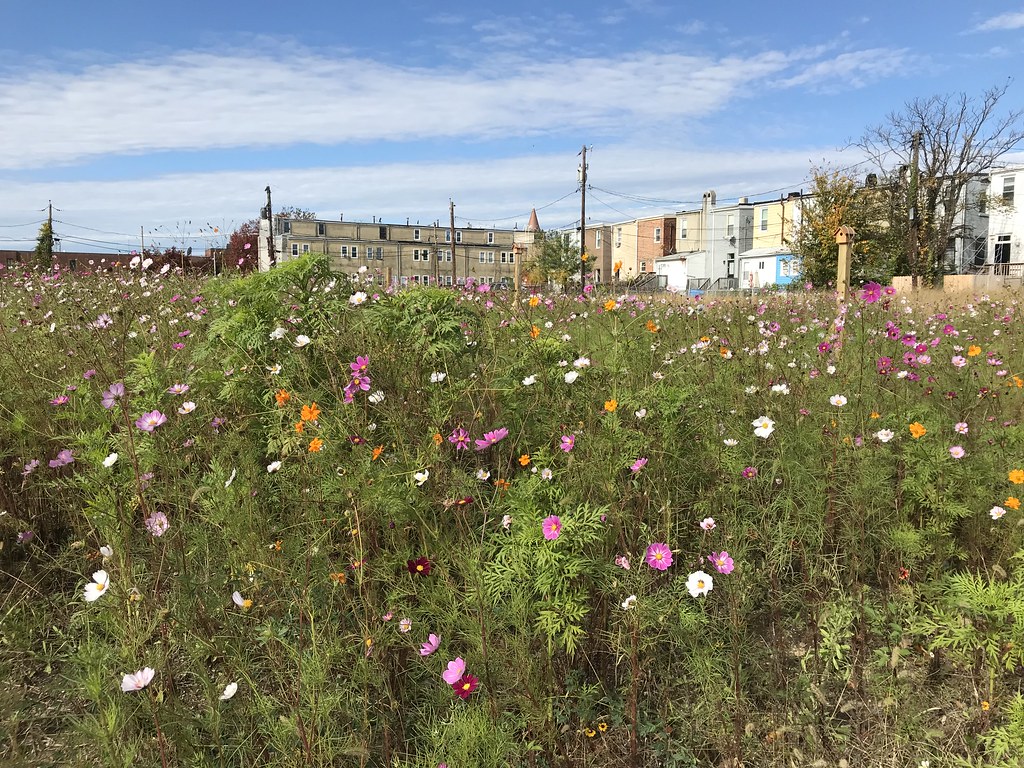A vibrant color photograph captures a lush field of wildflowers in the foreground, which takes up about two-thirds of the image. The flowers — predominantly pink, white, orange, purple, and yellow, with a few red ones — resemble various daisies and are interspersed within thick, thriving plant life, including some that appear fern-like. The field extends all the way to the horizon, where it meets a backdrop of row houses. These houses, with varied and colorful facades reminiscent of San Francisco architecture, are situated towards the left and center, with a larger, more prominent building near the left side. Utility poles with power lines stretch across the horizon from left to right, and in front of the houses, there are occasional trees and a birdhouse mounted on a post. Above, the blue sky features wispy white clouds, adding to the picturesque scene.